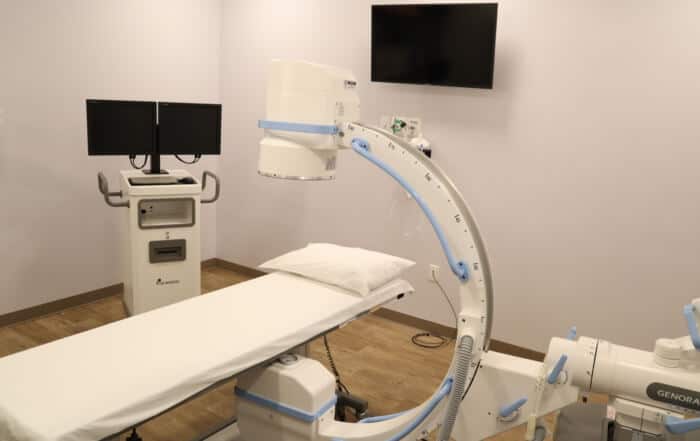The photograph captures the interior of a compact medical examination room, possibly in a hospital or clinic. The room features light gray walls on either side and a wooden tile floor with solid brown baseboards. Prominently positioned in the upper right corner is a flat-screen monitor mounted on the wall. Adjacent to this monitor is a white machine station with big gray handles, two blacked-out monitors, and additional components including a keyboard and a mouse. Centrally positioned, there is a narrow bed diagonally oriented from the lower left to the center of the image, complete with a small pillow. Suspended above the bed is a white, semi-circular machine with blue wires and various numbers marked on it. This intricate piece of equipment, possibly a lighting or scanning instrument, spans beneath and over the bed, enhancing the room's clinical feel.